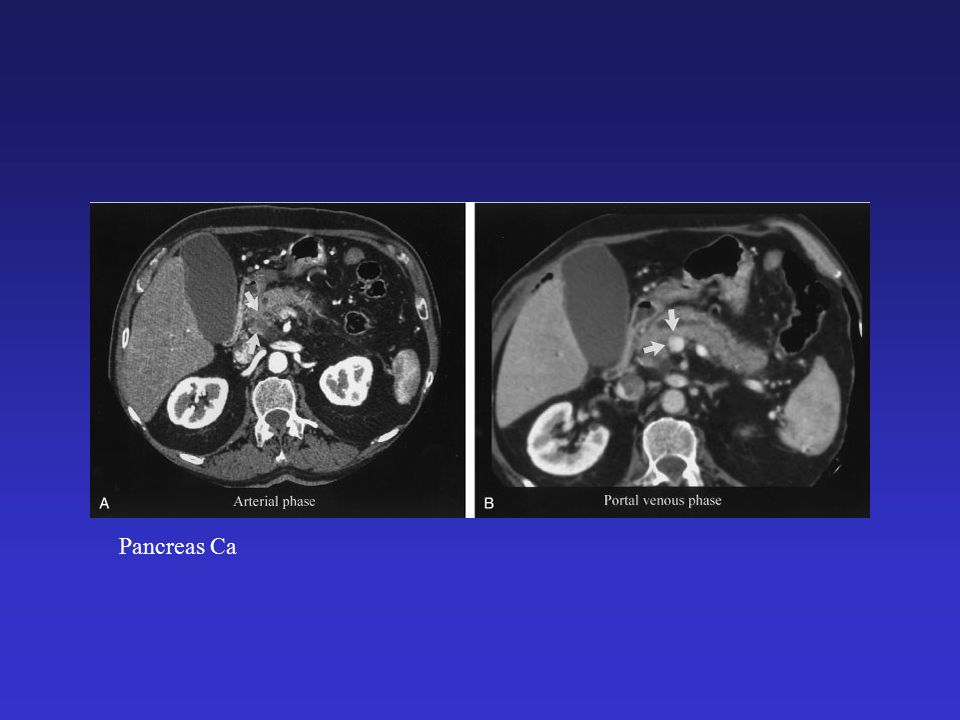The image displays two detailed cross-section scans of the pancreas, each distinctively labeled and positioned side by side against a gradient blue background that shifts from dark at the top to lighter at the bottom. On the left, the first scan is marked as "A" for the arterial phase, and on the right, the second scan is labeled "B" for the portal venous phase. Both scans are in black and white, and within them, arrows highlight specific areas—particularly in the arterial phase where arrows point to some matter at the center, and in the portal venous phase, where arrows indicate a white mass at the center of the scan. Below these images, in white font, the label "pancreas CA" signifies that the scans represent different phases of pancreatic imaging, possibly for educational or medical conference purposes.